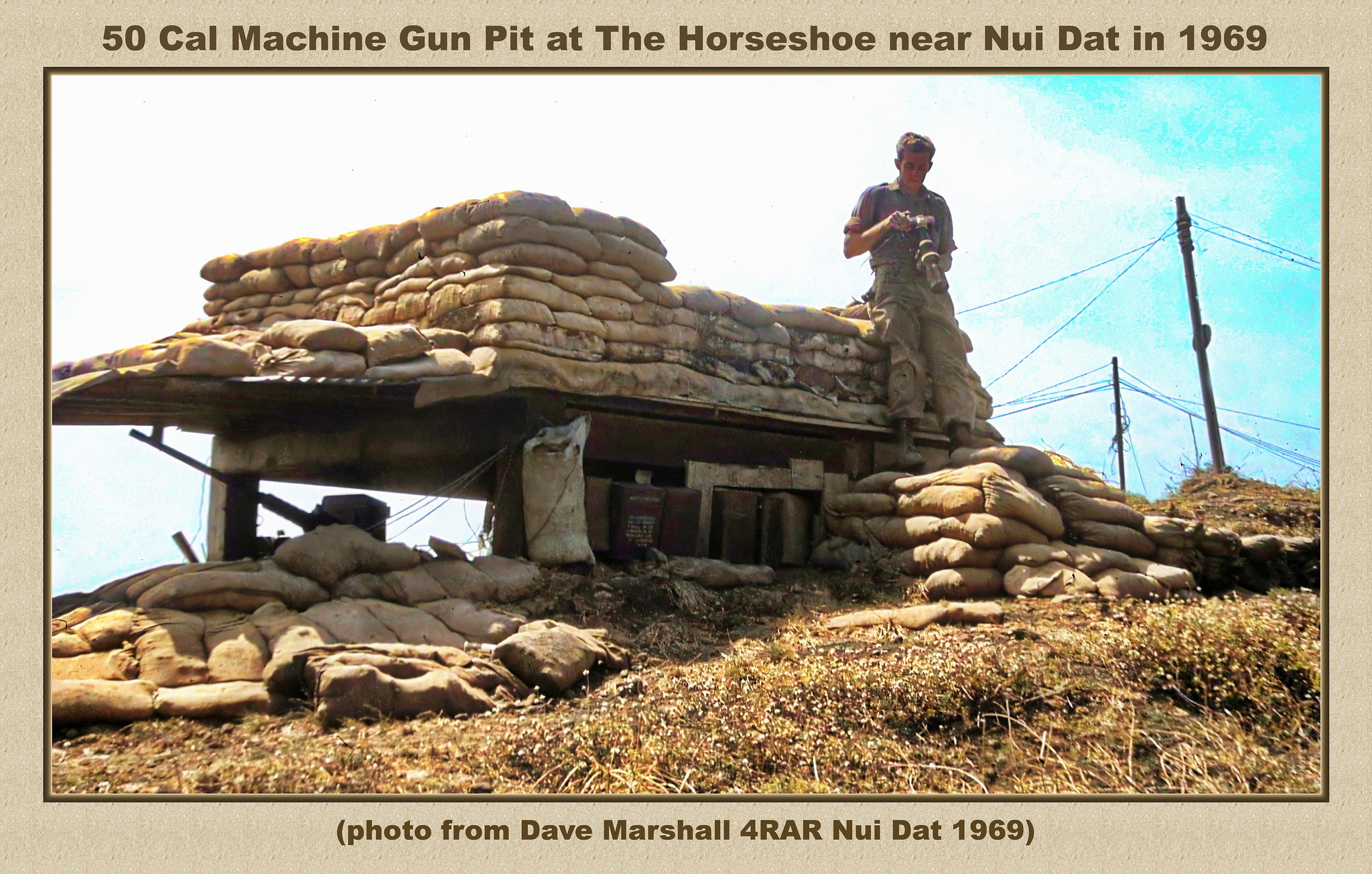This faded color photograph, taken outdoors during the daytime in 1969, captures a solitary photographer standing next to a fortified mound of sandbags at the Horseshoe near Nui Dat. The man, identified as Dave Marshall, holds a camera pointed downward. The sandbags, positioned on a dirt and grass hill, form a protective barrier around a .50 caliber machine gun, which is visible protruding from a dug-out pit. The background features a bright turquoise sky with wisps of clouds and visible telephone poles and wires. The image is captioned: "50 Cal Machine Gun Pit at the Horseshoe near Nui Dat in 1969," and credits the photo to Dave Marshall for RAR Nui Dat 1969.